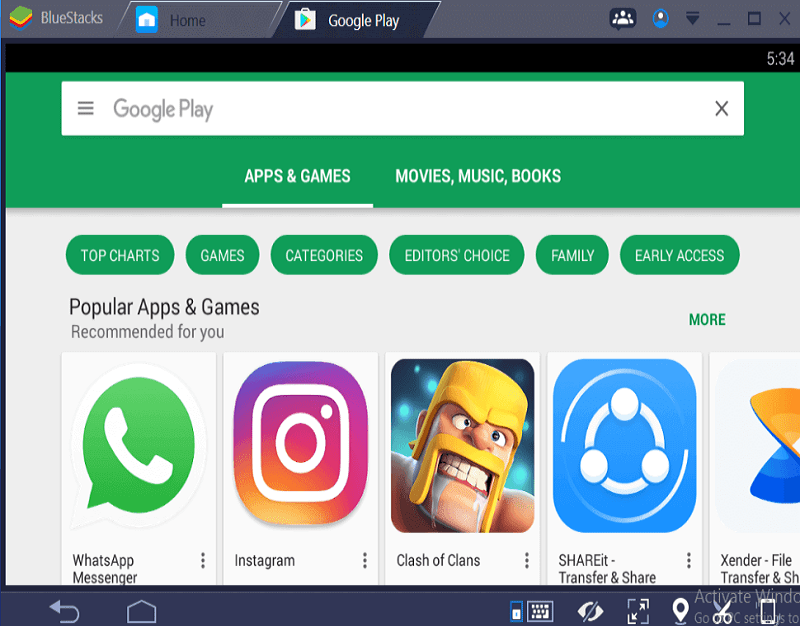The image depicts the Google Play Store interface on a device. The background is predominantly green, particularly noticeable at the top section. Centered within this area is a lengthy search bar with the text "Google Play" inside, accompanied by an 'X' on the right side of the bar. Below this, in white text, are the categories underlined in white: "Apps & Games," "Movies," "Music," and "Books." The time displayed on the device is 5:34.

At the top of the interface, several options are visible: "BlueStacks" (presumably an application), an icon resembling a stack of multi-colored books (green, yellow, red, and blue), "Home," and "Google Play." Nearby, there are green horizontal ovals with white text displaying categories such as Top Charts, Games, Categories, Editor's Choice, Family, and Early Access.

Beneath these options, the interface lists popular apps and games in black text with sections such as "Recommended for You." The apps featured include "WhatsApp Manager," "Instagram" with its recognizable purple and orange gradient square encompassing a camera image, "Clash of Clans" featuring an animated character with a gritty expression, a yellow helmet, and a square yellow mustache, and "SHAREit," represented by a blue square with a white circle inside.